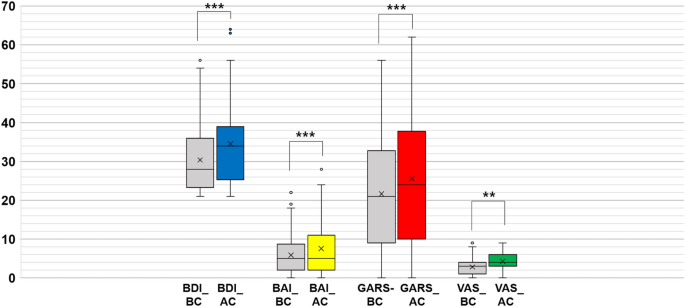The image depicts a wide, horizontally-oriented infographic, approximately three times wider than it is tall. This infographic showcases a bar graph featuring several vertical rectangles of different colors including gray, blue, red, yellow, and green. The vertical axis on the left is marked with numbers ranging from 0 to 70 in increments of 10. Horizontal lines intersect the graph, aligning with the numerical scale. The horizontal axis at the bottom is labeled with various acronyms such as BDI_BC, BDI_AC, BAI_BC, BAI_AC, GARS_BC, GARS_AC, VAS_BC, and VAS_AC, though their meanings are unspecified. The background of the infographic is white, and while the precise data or context is not clear, the graph visually organizes the information with colored bars corresponding to these acronyms.